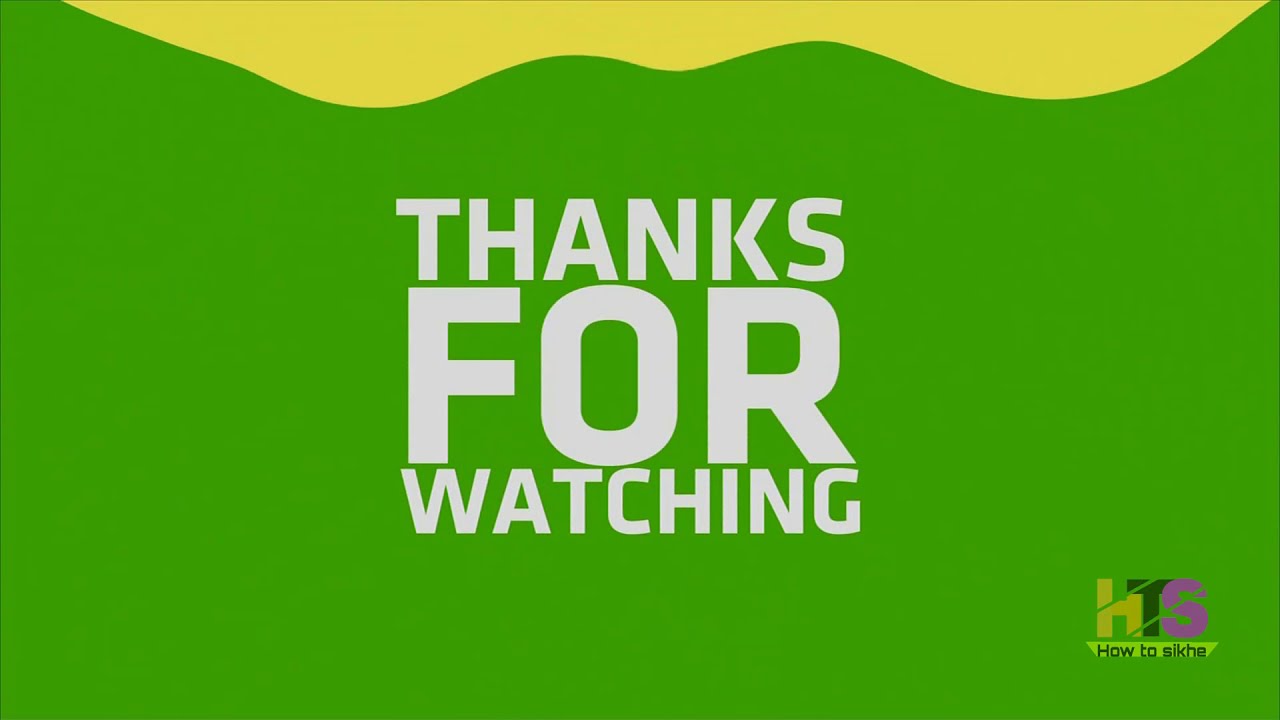The image appears to be a concluding screen for a video or TV show, featuring a predominant emerald green background. At the top 10% of the image, there is a wavy, mustard-yellow line. Centrally positioned in bold white letters, the text reads "Thanks for watching," with "Thanks" on the top line, "for" beneath it, and "watching" on the third line. In the bottom right corner, there is a small logo with the letters "HTS," accompanied by very small font letters spelling "S-I-K-H-E." Other notable details include a simplistic design reminiscent of the Sprite logo, utilizing a yellow and green color scheme.